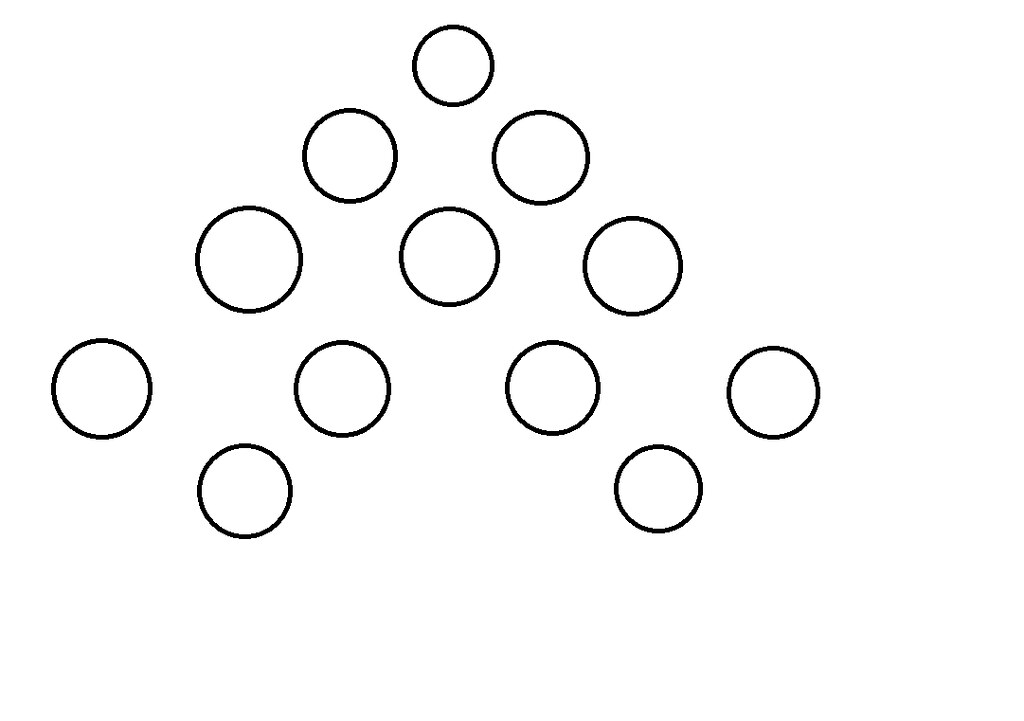This image appears to be a computer-generated graphic with a minimalist design featuring an array of black circles against a pure white backdrop. On the left side, there are four circles arranged diagonally, ascending to the right. These circles are mostly uniform in size, except for the top one, which is slightly smaller. Adjacent to this are four more circles, also forming a diagonal line upwards to the right, with each being equally sized. 

Following this, there's a row of just two circles, maintaining the same upward diagonal orientation. The final series features two circles that break the established pattern; while the first circle of this pair follows the diagonal alignment, the second one is misaligned, jutting off to the right. None of the circles overlap or touch each other, and they are irregularly spaced, contributing to a sense of disarray in their arrangement. This entire black-and-white composition emphasizes the stark contrast and deliberate misalignment of its elements.